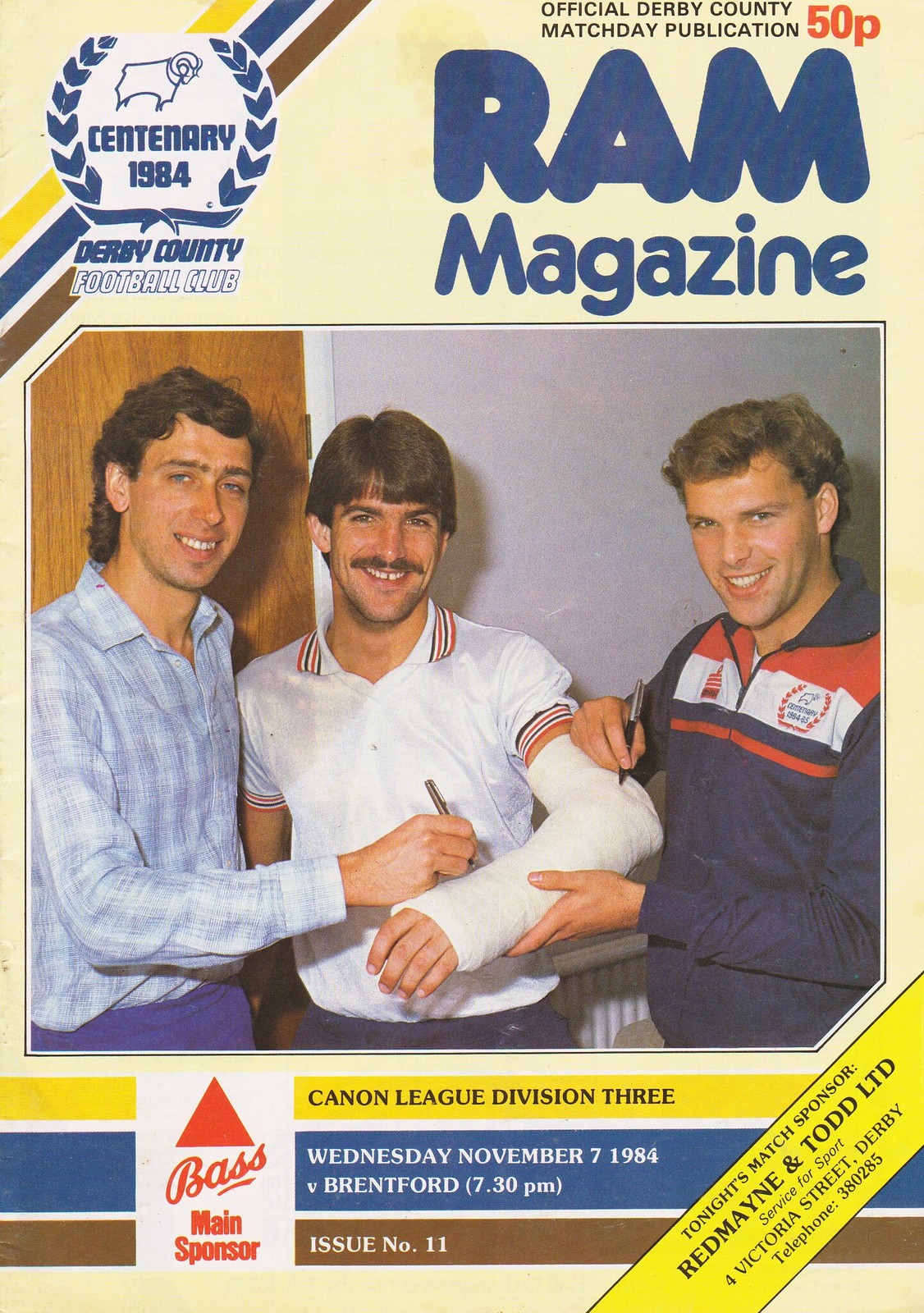The cover of RAM Magazine, dated Wednesday, November 7, 1984, prominently features a photograph of three Caucasian men in their 20s or 30s. The man in the center, wearing a white polo shirt, has a white cast on his left arm and sports brown hair and a mustache. He is flanked by two men holding markers, presumably about to sign his cast; the man on the left has black hair and a blue-toned button-up shirt, while the man on the right wears a zipped-up jacket and has short brown hair. All are smiling directly at the camera against a light gray background with a wooden door visible on the left.

The top of the magazine bears the title "RAM Magazine" in dark blue, accompanied by the Derby County Football Club logo featuring a white ram with a blue border, overlayed text reading "Centenary 1984," and "Derby County Football Club" in blue and white. Further details include the issue number (11) and specifics about the match: "Cannon League Division 3, Wednesday, November 7, 1984, V Brentford 7.30 p.m."

Additional elements include a red and white Bass logo noting the main sponsor, displayed at the bottom of the page. A yellow ribbon in the lower right corner mentions tonight's match sponsor, "Red Main and Todd LTD, service for sport, Victoria Street, Derby, telephone 380285," in black text. The color scheme prominently features blue, white, yellow, and brown, chronicling a nostalgic piece from mid-1980s football culture.